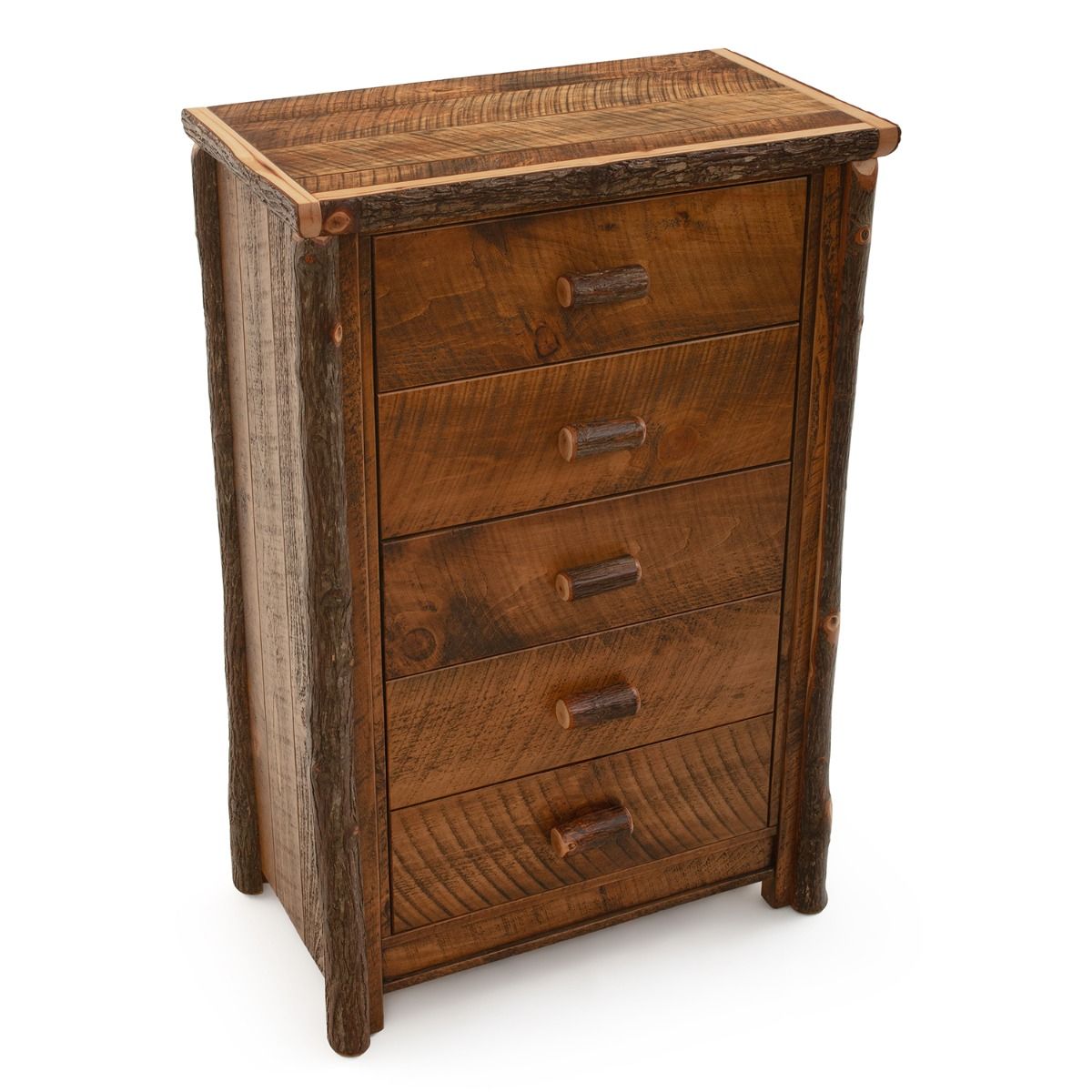This image showcases a rustic, five-drawer dresser made from dark wood with visible grains and a handcrafted finish. The dresser is photographed against a pristine, white background, typical of a retail website, with a slight angle that reveals the front, part of the side, and the top. The wood retains its natural appearance, although there's an artful interplay between human finishing and natural elements. This is evident from the grain patterns and the unique stripes introduced during varnishing. 

The dresser features log section handles on the drawer fronts, in addition to cylindrical, unrefined wood legs at each corner, enhancing its rugged aesthetic. The dresser's flat top incorporates similarly crafted log elements around its edges, yet the top surface itself remains smoothly finished. Each of the five drawers is closed, leaving the internal structure to the imagination. The piece casts a subtle shadow beneath it, adding to its three-dimensional presence in the image. The tops of the dresser and its sides show varying shades of brown, with the top being slightly lighter, enhancing the texture and depth of the woodwork.